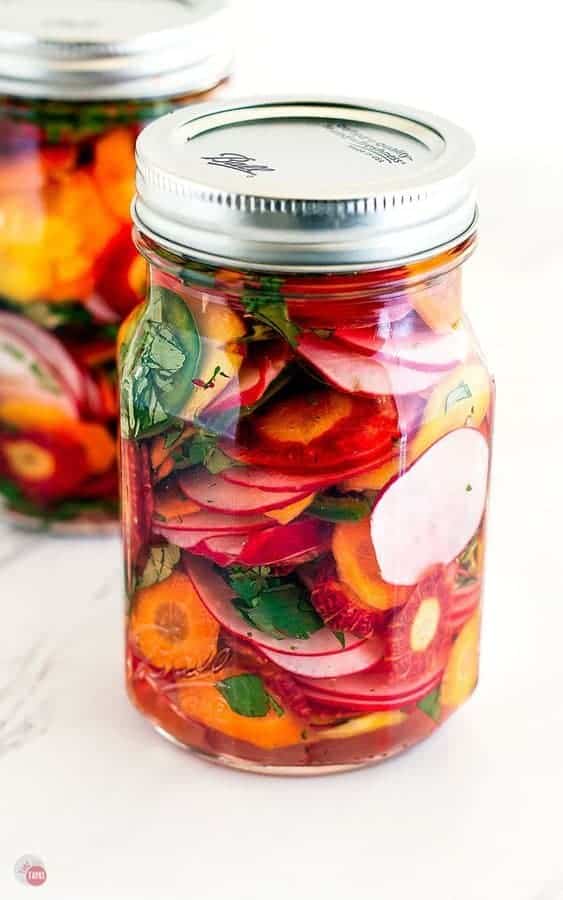This image features two clear jars with metal lids, prominently placed on a marble-like table. The jar in the foreground is in sharp focus, displaying a colorful assortment of thinly sliced fruits and vegetables immersed in liquid. The vividly detailed contents include slices of radishes, carrots, sweet potatoes, tomatoes, lemons, red onions, and green leaves that likely include cilantro. The jars appear to be pickling these items. The background features a second, blurred jar placed at the top left, mirroring the contents of the primary jar. Both lids are metallic and branded, presumably with the popular "Ball" logo. The scene is set against a white background, making the vibrant colors of the jarred ingredients stand out.